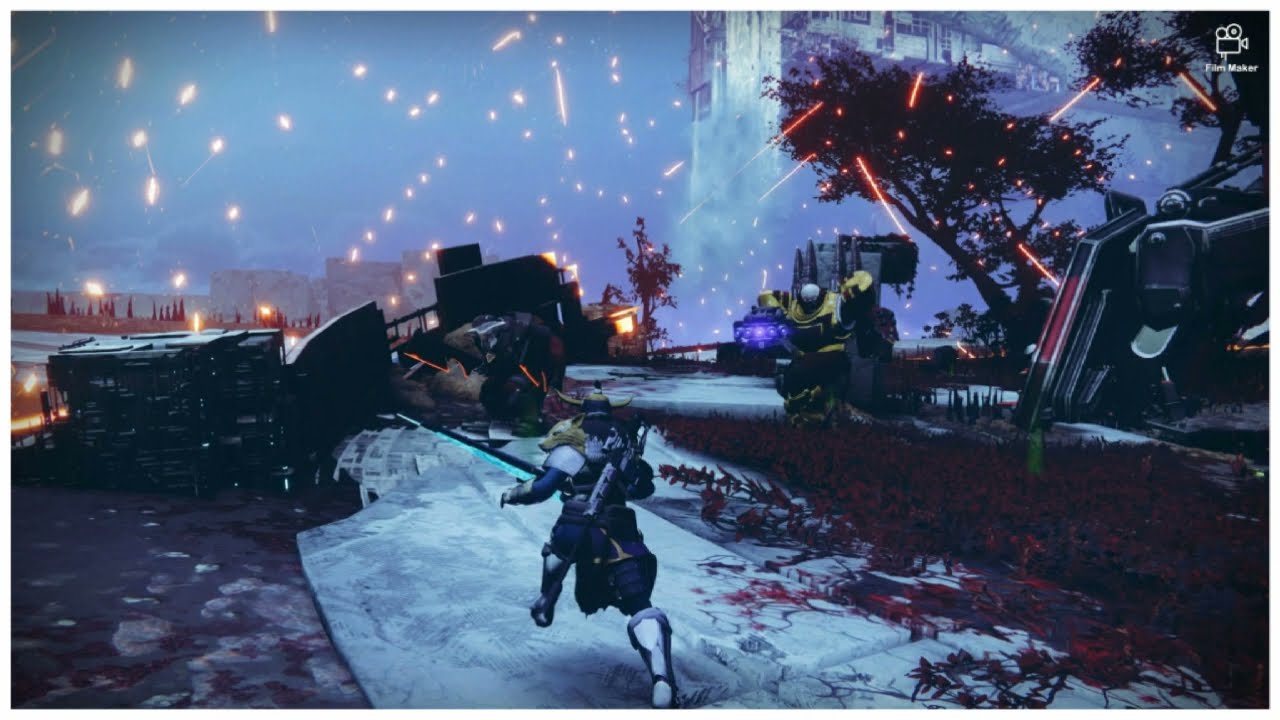In the midst of a chaotic battlefield, set within a scenic yet devastated landscape, our focus is drawn to a central character decked out in dark navy blue and white armor. This solitary figure is running in the 11 o'clock direction, striding atop what appears to be the wing of a crashed airplane, surrounded by scattered debris of destruction. The character carries a silvery gun strapped to his back and is navigating through an environment rife with peril. The sky above is a stark light blue adorned with dark purple clouds, hinting at a recent or ongoing conflict. 

All around, bullets and streaks of fire arc through the air, their trajectory forming orange trails that illuminate the chaotic scene. At least 10 to 15 guns are being fired, though, fortunately, none of the bullets seem to be aimed at our central figure. To the right, another figure in gold armor stands out among the destruction, potential adversaries in the making. The ground beneath is littered with maroon streaks, possibly blood or charred earth, while the trees and futuristic structures in the background bear the scars of the ongoing battle with explosions and artillery flashes highlighting their ominous silhouettes. In the top right of the scene, there's a glaring white and purple building, adding to the desolate ambiance of this war-torn environment.